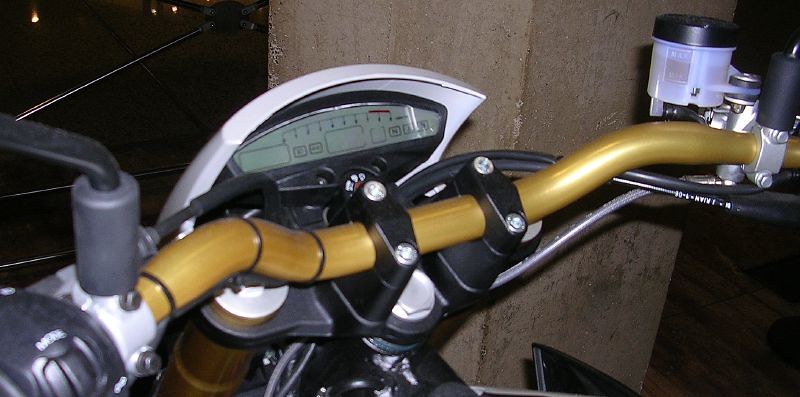This photograph captures a close-up view of a motorcycle’s handlebars and dashboard area, highlighting the intricate details of its design. The handlebars are a striking gold color and stretch across the entire front top section of the motorcycle. They are securely mounted to the body of the motorcycle using black brackets fastened with silver screws. Just above the handlebars, there is a prominent gauge with a silver arch at the top and a clear plastic covering, though the exact details on the gauge's face are not legible. The base of the handlebars, where they connect to the motorcycle’s body, is predominantly black and features some gray wires emerging from the left side. Extending from the ends of the handlebars are hand brakes, combining gray and black elements for a cohesive design. This detailed view provides an intimate look at the mechanics and aesthetics of the motorcycle’s control area.